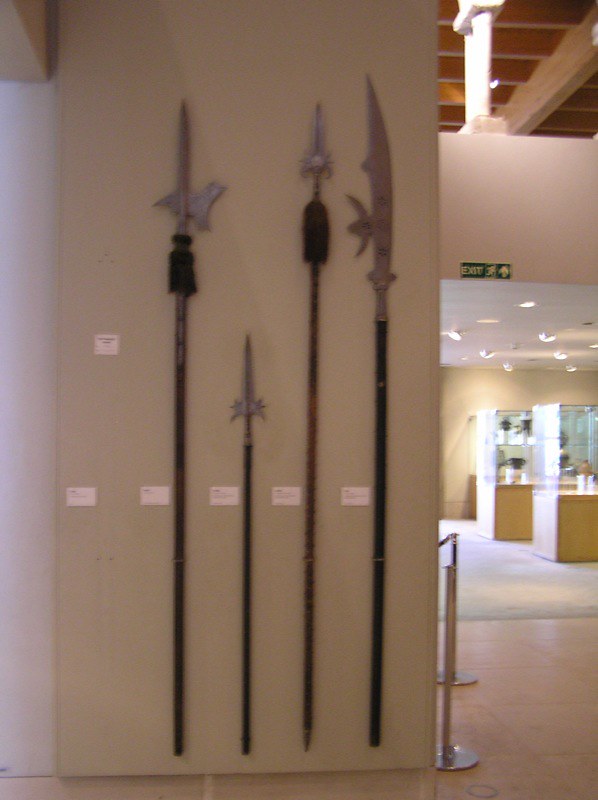The image is a blurry vertical photograph taken in a museum where flash photography is likely discouraged. The focal point of the image is a display on a beige wall showcasing a collection of medieval or renaissance-style weapons. There are labels next to each weapon, but the blur renders them unreadable. Among the displayed armaments, there is a spiked long halberd, a very short spear, a long tasseled spear, and a naginata, a Japanese long polearm with a machete-like blade. The weapons are mostly in darker hues such as brown, black, and silver. In the background, there are indistinct glass cases holding various objects, further suggesting the setting to be a museum or gallery.